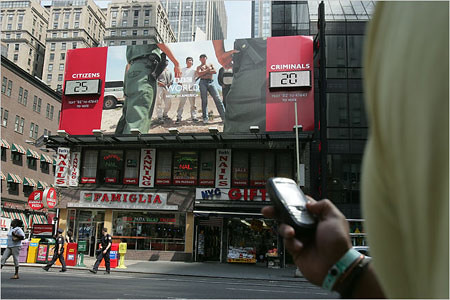A person is partially visible in this image, specifically from the chest area and torso on the right side, which is cut off midway. The individual is slightly turned to the upper left, holding a small cell phone in their right hand. An aqua wristband adorns the wrist holding the phone. In the background, a city skyline is visible, characterized by tall buildings. A prominent billboard stands atop a two-story business. The billboard features images of four people, including two policemen facing away from the camera. The left side of the billboard displays the word "Citizens" alongside a digital screen showing the number 25, while the right side displays "Criminals" with a screen showing the number 20.